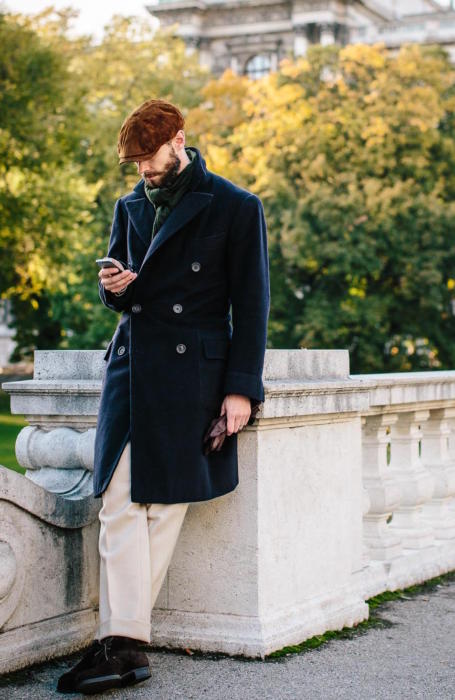In this detailed outdoor photograph, a man stands slightly to the left of center on a stone or concrete walkway, leaning against a white stone railing. He is dressed in dark shoes, white pants, and a buttoned-up, knee-length navy blue overcoat, suggesting a slightly chilly day. He holds a pair of gloves in his left hand, which hangs down at his side, and in his right hand, he looks down at an older model phone. His brown flat cap, pulled low, conceals his eyes, and he has a full beard and mustache. The background features blurry green trees with sunlight reflecting off them, giving a hint of brightness to the scene. A large stone building is partially visible beyond the trees, adding to the professional quality of the photograph. The white sky suggests the photo was taken during daylight.